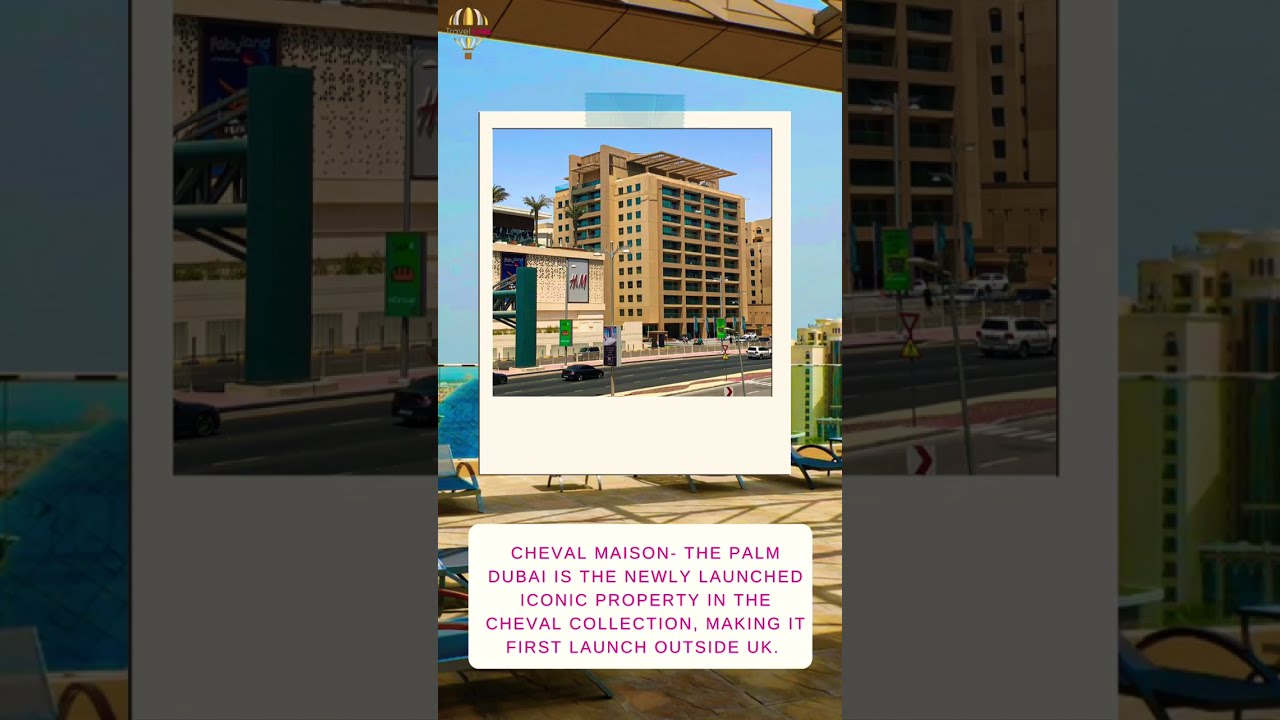The image showcases an advertising display for a newly launched property called “Cheval Maison, The Palm Dubai,” part of the Cheval collection, and marks its first launch outside the UK. The display itself is a photograph of an artist's rendition designed to look like a Polaroid snapshot and features a tan-colored, multi-story high-rise building, possibly a hotel or condominium, with at least 11-12 stories. This main building, illustrated to appear complete, has numerous windows and tiered openings, with an overhang suggesting an outdoor area at the top. Slightly shorter buildings flank the main structure. 

The foreground announces "Cheval Maison" in purple, uppercase lettering within a white box. Notably, the image composition is a picture within a picture: the central strip focuses on the building, flanked by darker, zoomed-in fragments of the same image, which makes up the majority of the frame. A black concrete road with a few cars runs in front of the building, hinting at an active street scene. Beyond the building, palm trees are visible against a clear blue sky, enhancing the idyllic, resort-like feel of the property.